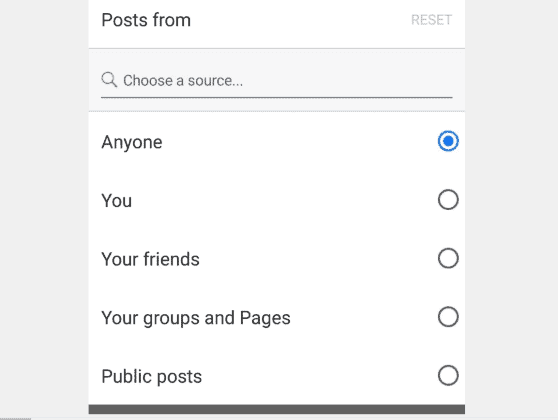The image depicts a user interface element, likely from a social media platform. It features a square with very light gray shading, creating a margin a couple of inches in from each side. Within this margin is a white square area.

Starting from the left of this white square, there is the text "Post from," with "Post" having a capital 'P' and written in a darker black script. To the right, on the edge, there is the term "Reset," displayed in a lighter gray font.

Below this text row, there is a shaded square containing a magnifying glass icon, and next to it, the instruction "Choose a source," with only the 'C' capitalized.

Following this, there are several selectable options denoted by circular radio buttons:

1. "Anyone" - written in a darker font with a blue circle in the middle, indicating it is the currently selected option.
2. "Your Friends" - the 'Y' in "Your" is capitalized.
3. "Your Groups and Pages" - both 'Y' in "Your" and 'P' in "Pages" are capitalized.
4. "Public Posts" - the 'P' in "Public" is capitalized.

At the bottom, there is a thicker border running across the entire width of the interface, emphasizing the end of this section.